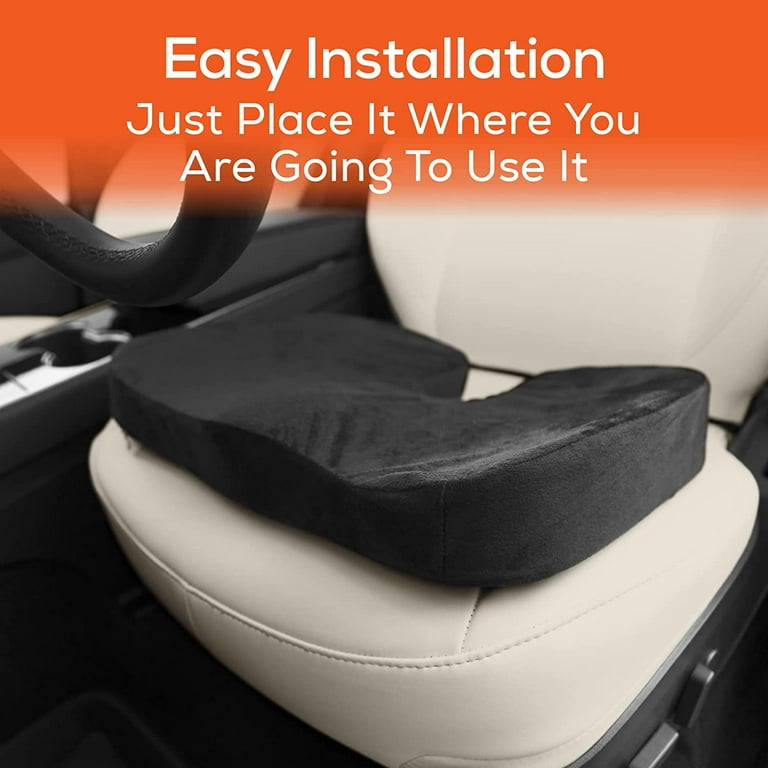This image is a detailed product advertisement for a portable, contoured seat cushion designed for easy installation in a car. The scene focuses on the driver's seat of a car, featuring a cream-colored, leather front seat with visible seat adjustment levers on the side. Draped over the seat is a thick, black U-shaped cushion, made from a fuzzy, velour-like material. This cushion is notable for its ergonomic design, specifically its tailbone cut-out to provide comfort and alleviate pressure. Above the seat, an orange band prominently displays the text "Easy installation, just place it where you are going to use it," emphasizing the product's portability and versatility for use in various seating situations, whether behind your back, underneath you, or around your neck. The bottom half of the steering wheel is visible, reinforcing that this is indeed an automotive context, enhancing the cushion's appeal for car use.